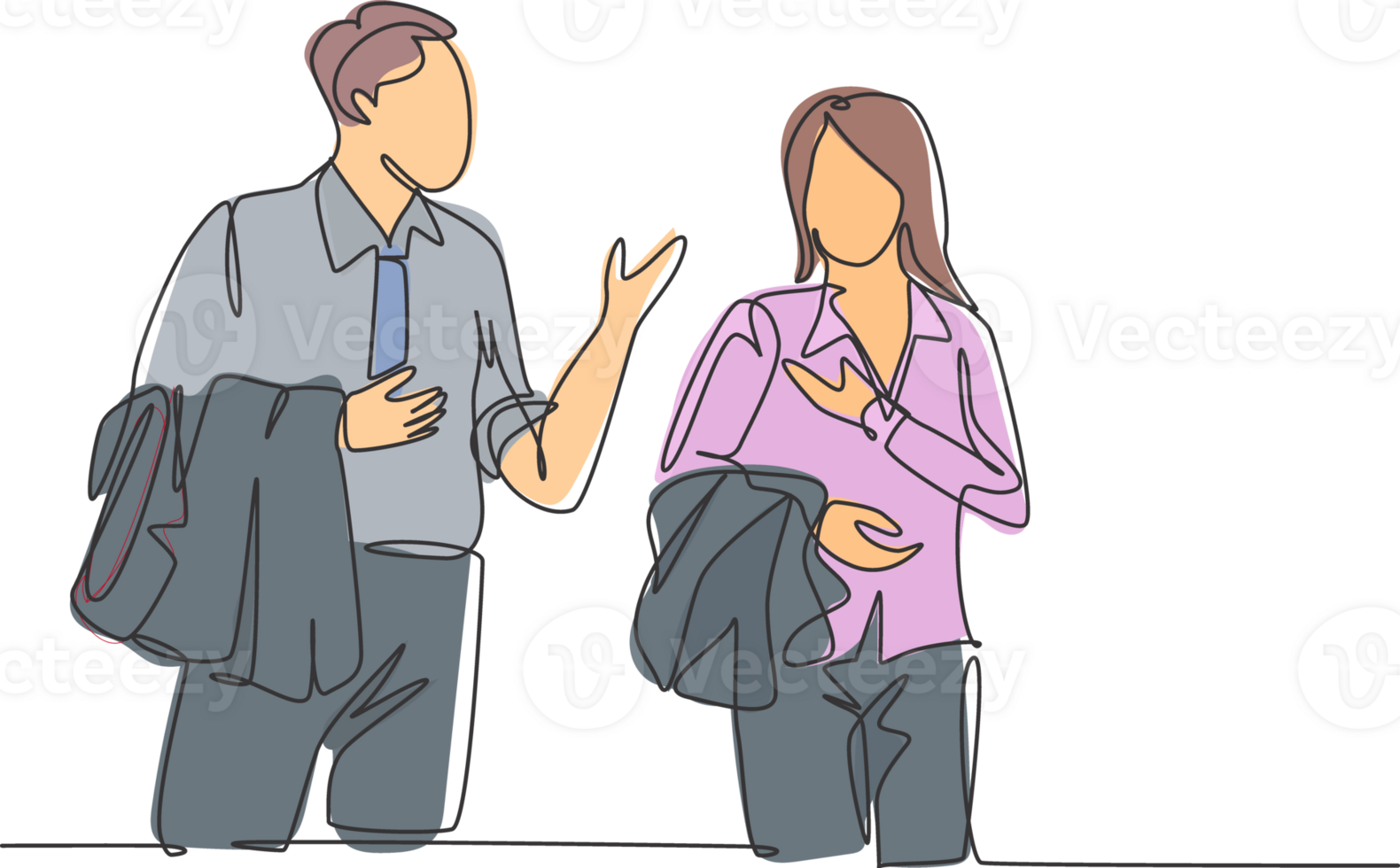This illustration depicts a man and a woman standing side by side, engaged in conversation. They both have brown hair; the man's is short, while the woman's reaches her shoulders. Neither character has facial details, presenting blank faces with only chin and necklines visible. The man, standing on the left, wears a grey shirt paired with a blue tie and grey slacks, mirroring the woman's attire, which consists of a light violet business shirt and similar grey trousers. Both are holding their matching grey jackets draped over their left arms. The rough, curved lines and colored pen style contribute to the simplistic, almost sketch-like quality of the illustration. The man appears to gesticulate with his right arm as he speaks, and the woman’s right hand is also raised, possibly responding in the gesture-filled dialogue. The scene suggests a moment after work, given their relaxed handling of their jackets. The woman’s slightly darker tan contrasts subtly with the man’s lighter complexion.